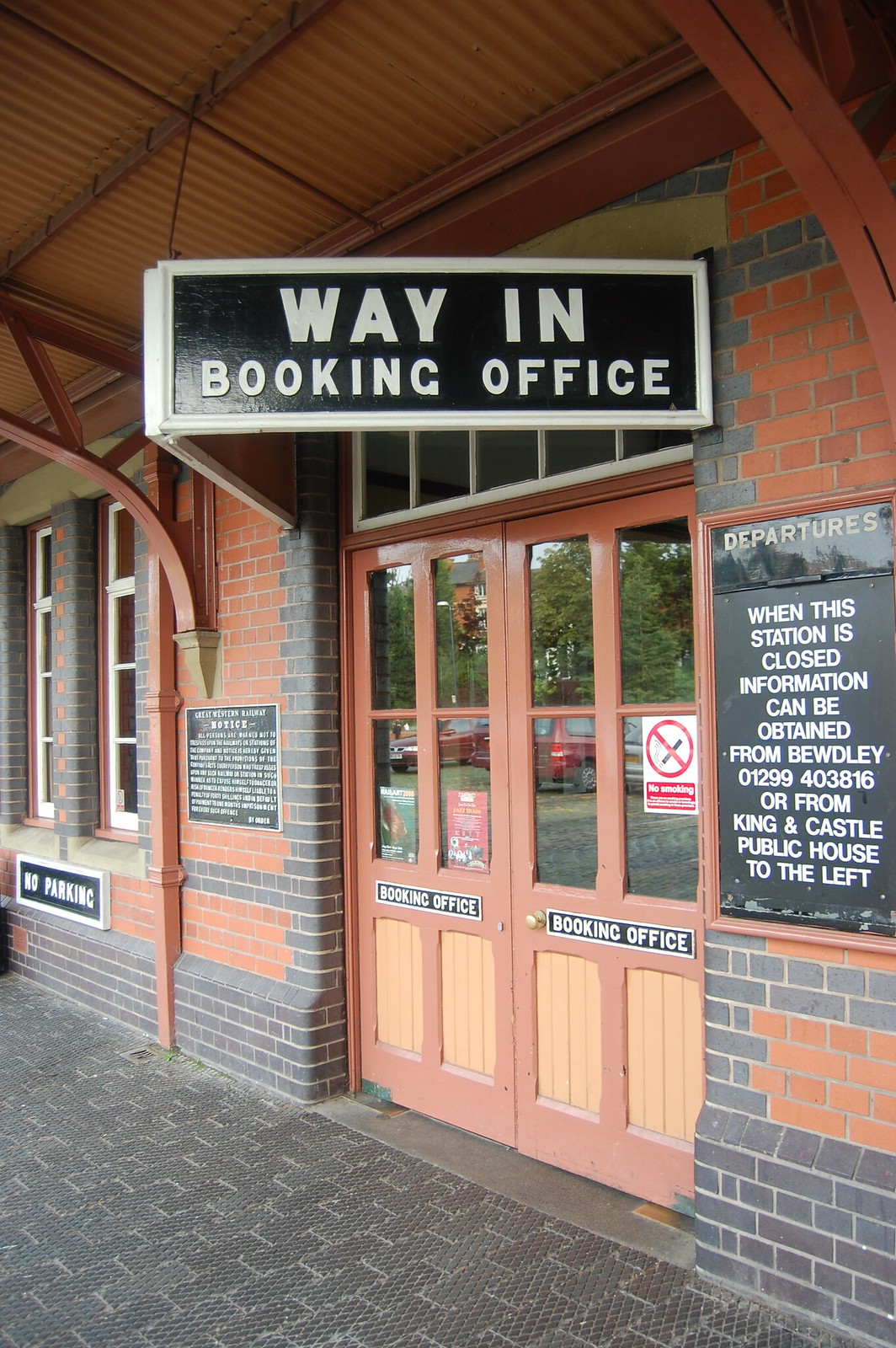The photograph depicts the entrance of a booking office set within a brick building, showcasing both red and gray brickwork. The building features arched supports that hold a metal-covered walkway, providing shelter above two large wooden double doors. Each door is adorned with four double-pane glass windows, with the words "Booking Office" inscribed beneath them. A triangular sign, visible from both sides, extends above the entryway, displaying "Way In Booking Office" in white text on a black background with a white border.

To the far left, there's a prominent black sign bordered in white that reads "No Parking." On the right side of the doors, another large sign labeled "Departures" is posted. Below this departures sign, information is provided detailing that, when the station is closed, details can be obtained from the Woolley or from the King and Castle Public House.

The lower right pane of the door holds a "No Smoking" sign, while posters, difficult to discern, adorn the other lower panes. The sidewalk in front consists of rectangular gray pavers, completing the office’s inviting entrance.